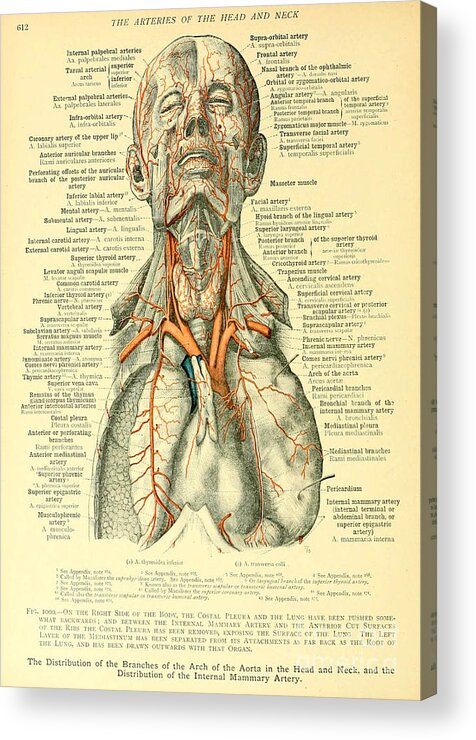This vertical rectangular image resembles a medical reference chart, potentially a poster or a page from a thick book. The chart is primarily yellow or beige and appears to be slightly turned away from the viewer. Dominating the visual is a detailed anatomical diagram featuring a man’s head, neck, and upper torso, with his lungs and heart exposed, devoid of any skin or rib coverage. The man's body has a greenish tinge, contributing to a somewhat eerie appearance.

The central diagram intricately highlights the arterial system, showcasing a network of orange and red lines representing arteries, capillaries, and veins. These lines vary in thickness and are meticulously labeled, with annotations running down both sides of the diagram. Despite the abundance of text, the writing is too small to be deciphered clearly.

At the top of the chart, the title reads "The Arteries of the Head and Neck." Additional text is scattered throughout the image, with a notable section of barely legible, smaller writing at the bottom, which includes terms like "the distribution of the branches of the arch of the aorta in the head and neck" and "the distribution of the internal mammary artery." This detailed imagery and extensive labeling aim to convey a comprehensive understanding of the arterial structures within the head and neck, albeit in a visually dense and somewhat unsettling manner.